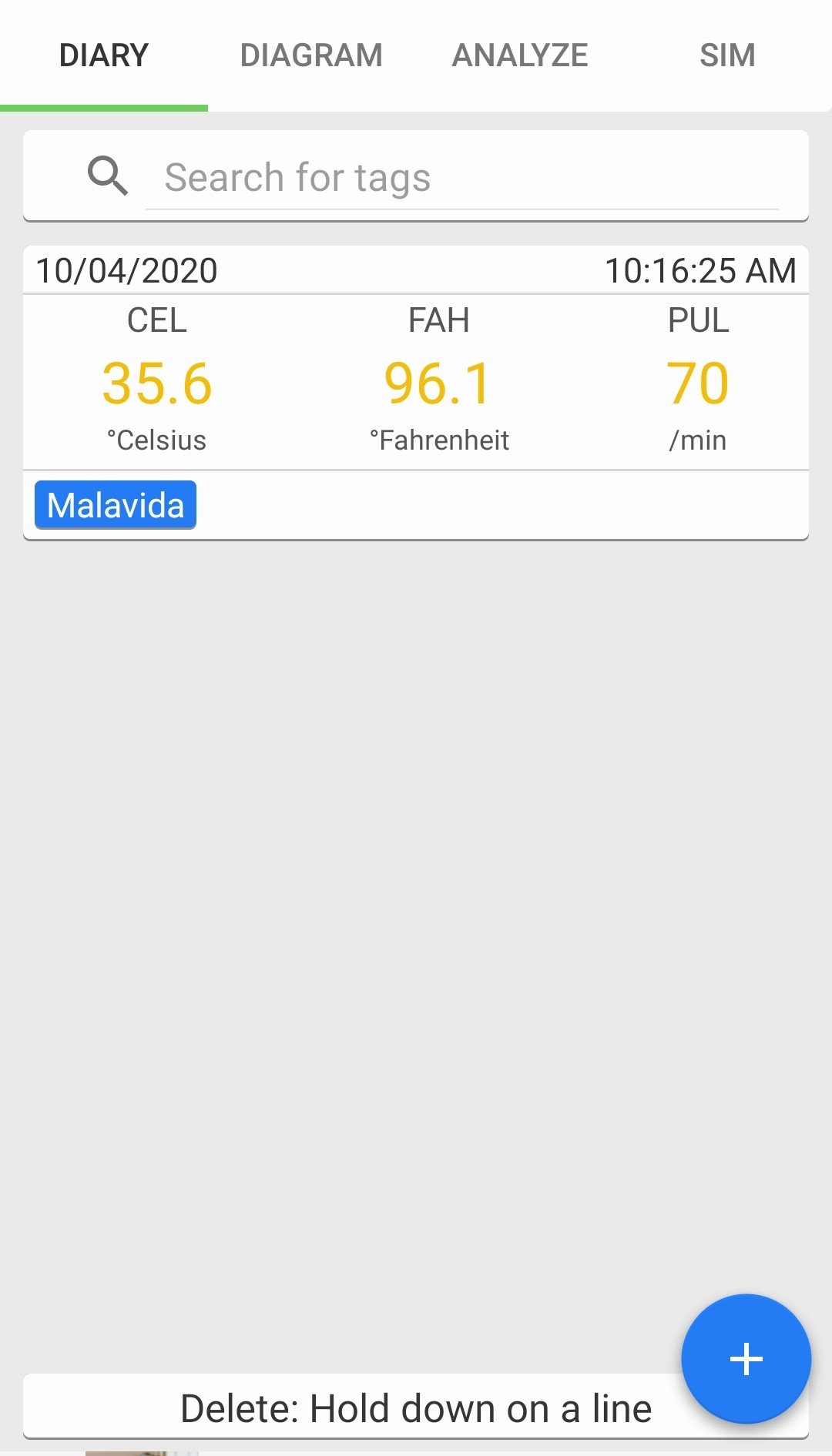This image is a detailed screenshot from a smartphone, taken in a well-lit environment. At the top of the screen, there is a light banner featuring four options in white or light gray text. The first option, "Diary," is highlighted in black text with a green underline, indicating it is currently selected. The other three options, "Diagram," "Analyze," and "Sim," are displayed in gray text. Below this banner, on a gray background, there are two white boxes.

The first box is a search bar with a search icon, containing the placeholder text "Search for Tags" in gray. Directly below the search bar is another box displaying a timestamp: "10/04/2020, 10:16:25 AM," separated by a gray line. This box also includes various health metrics: "CEL 35.6" in yellow text followed by "degrees Celsius" in smaller gray text, "FAH 96.1" in yellow text followed by "degrees Fahrenheit" in gray text, and "PUL 70" in yellow text followed by "/min" in smaller gray text. These metrics are divided by gray separator lines.

Underneath these metrics, there is a blue button with white text labeled "Malavida." Below the button lies an expanse of gray empty space, and at the bottom of the screen, there is a white box with black text advising, "Delete, hold down on a line." In the bottom right corner of the screen, a blue circle bears a white plus sign, presumably for adding a new item or widget to the page.